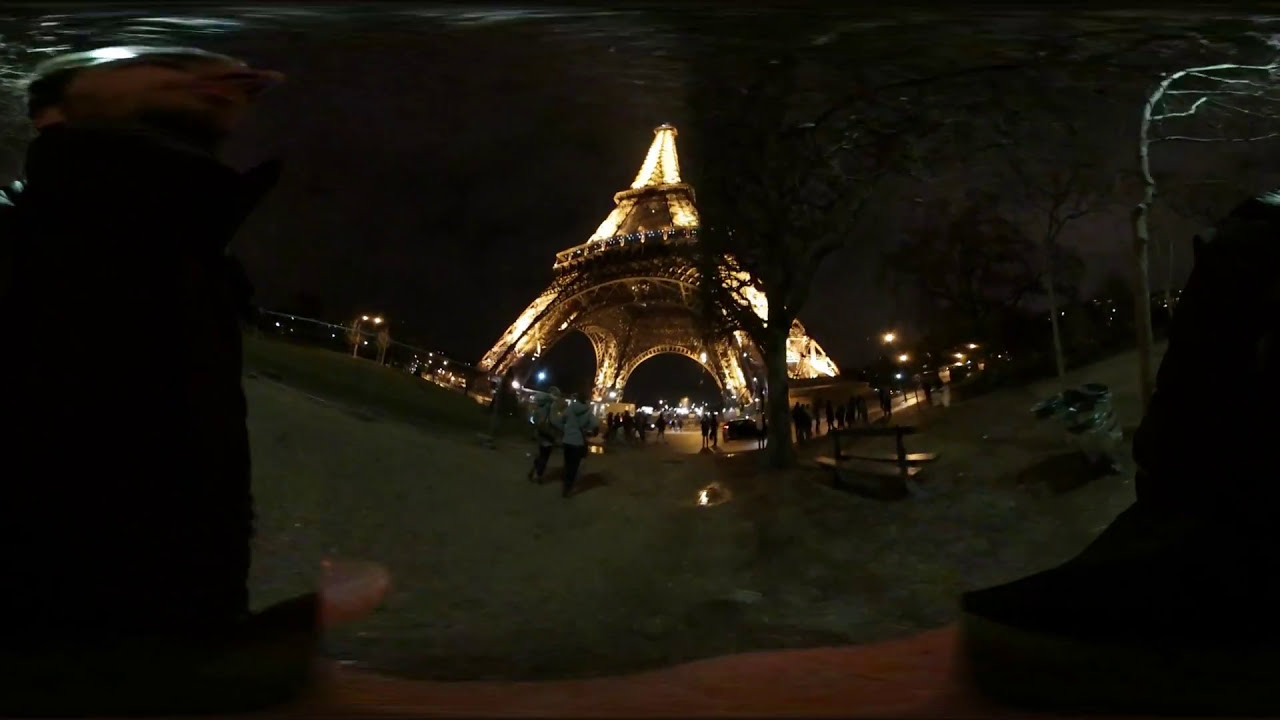This nighttime panoramic image, likely taken with a 360-degree lens causing fisheye distortion, centers on the brightly illuminated Eiffel Tower in Paris, casting a golden-yellow glow. The night sky is pitch black, making the tower's lights even more striking. A shadowy tree partially obscures the tower in the foreground, while other faint tree shadows are visible at both sides. The ground has a greenish-gray hue due to the indirect lighting from the tower.

In the medium foreground, several individuals can be seen, with many more people further back towards the tower, all dressed in winter clothing like jackets, long pants, and hats. The image features some vertical dark structures on the left and right, likely due to the panoramic stitching, giving the effect that the person taking the photograph appears on both sides of the image. Beneath a tree to the right of the center, there's a visible bench, enhancing the park setting that surrounds the tower. The scene captures a lively yet serene moment in a bustling city under the brilliance of one of its most iconic landmarks.